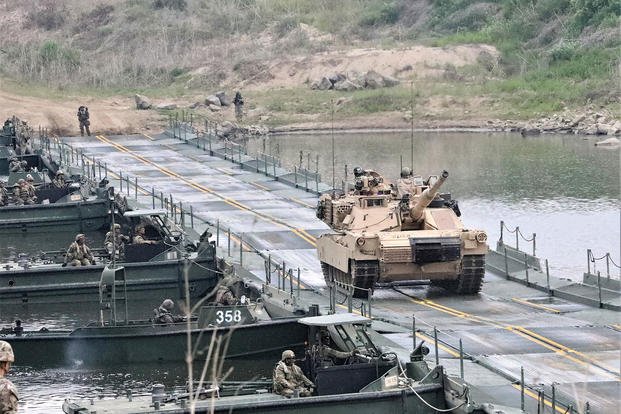The image captures a heavily-built, makeshift military pier extending across a calm lake, set against a backdrop of hills and rugged, scrub-covered terrain. The temporary structure, appearing unevenly pieced together, supports a tan military tank driving steadily along its length. At the end of the pier, a small group of soldiers stands watch. On the left side of the pier, five military pontoon boats, each fashioned in dark army gray, are moored with numbers like 358 visible on one of them. These boats, carrying two to four military personnel each, appear to be monitoring the tank's passage. The scene is framed by the stark contrast between the orderly line of boats and the serene, expansive waters on the opposite side of the pier.